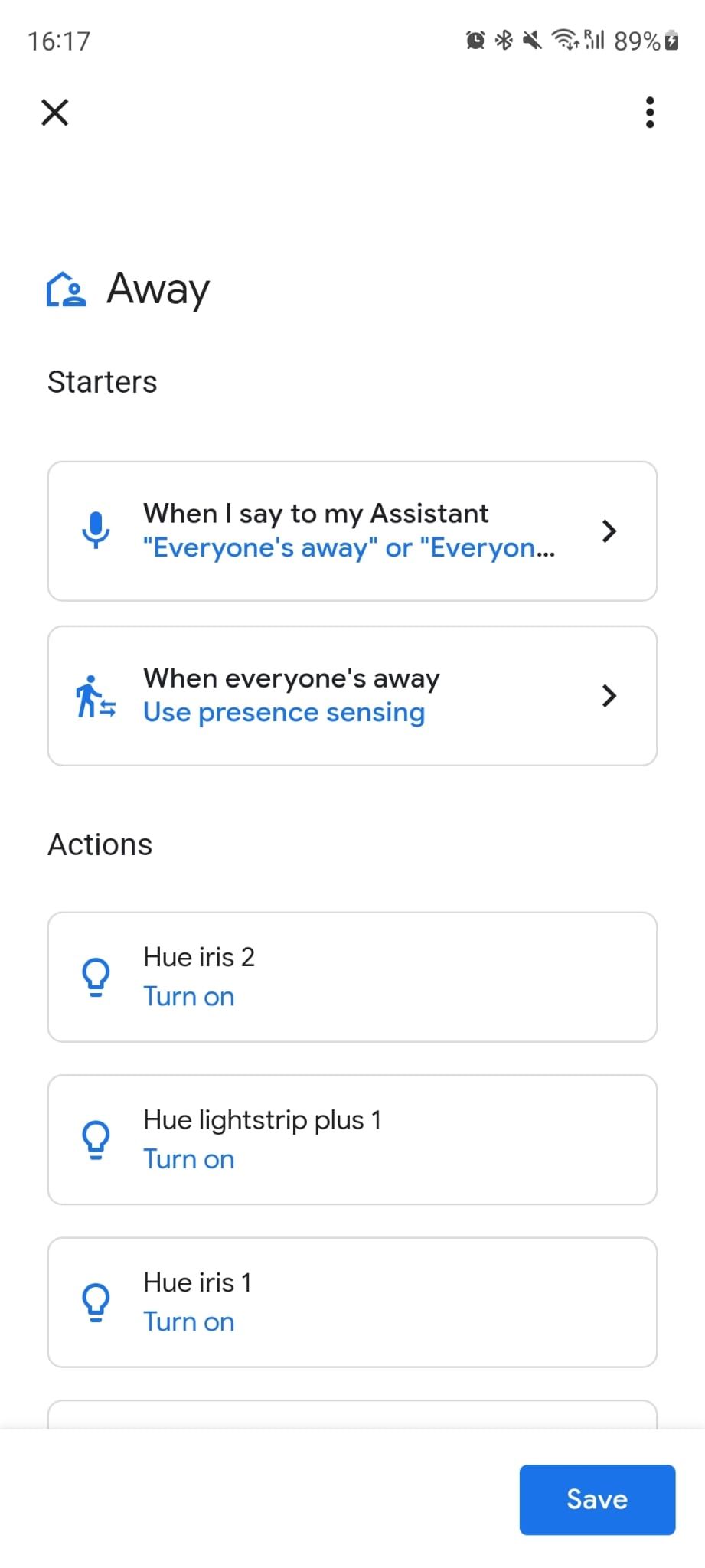The image is a screenshot of another mobile device featuring a predominantly white background with black and blue text. At the top of the screen, in black text, is the number "1617" followed by an array of icons on the right: an alarm clock, Bluetooth, silent mode, Wi-Fi strength, full signal, and an 89% battery indicator with a vertical battery icon. Just beneath these icons, on the left, is a black "X" symbol, and on the far right are three vertical dots.

In the center of the screen, prominently displayed, is the word "Away" in black text with a small blue icon to its left. Below this header is the word "Starters" in black. There are two interactive boxes beneath this section. The first box features a blue microphone icon and the text "When I say to my assistant" in black, followed by "everyone's away" or "everyone" in blue, accompanied by an arrow. The second box displays a blue walking man logo with the text "When everyone's away" in black and "use presence sensor" in blue, also accompanied by an arrow.

Further down under the "Actions" section in black text, there are three boxes each starting with a blue light bulb icon. The first box reads "Hue Iris 2" in black and "turn on" in blue beneath it. The second box states "Hue Lightstrip Plus 1" in black with "turn on" in blue below. The third box labels "Hue Iris 1" in black, with "turn on" written in blue text beneath it.

Finally, at the bottom right corner of the screen, there's a blue box with the text "Save" written in white.